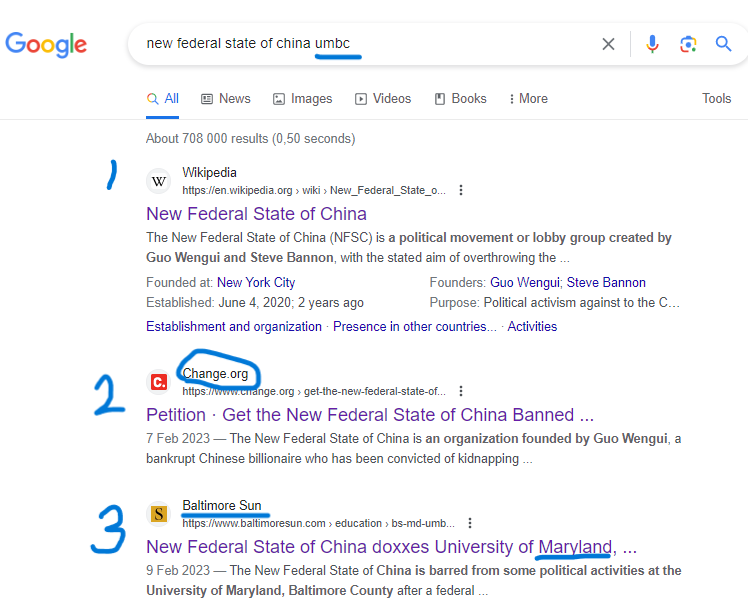The image depicts a Google web search results page with the query "New Federal State of China UMBC" entered into the search bar. At the top, the distinctive Google logo is prominently displayed, followed by the search bar containing the search query. To the right of the search bar are various icons: an "X" for clearing the query, the Google microphone for voice searches, the Google Image Search logo, and a magnifying glass icon for initiating the search.

Below the search bar, there's a row of tabs for filtering search results: "All" accompanied by a magnifying glass icon, "News" with a newspaper icon, "Images" with an image icon, "Videos" with a play button icon, "Books" with a bookmark icon, and "More" with three dots. To the far right, there's a "Tools" option.

The search results indicate approximately 708,000 results retrieved in 0.50 seconds. The first result is a link to Wikipedia with the URL "https://en.wikipedia.org/wiki/New_Federal_State_of_China," displayed in abbreviated form. The page title is highlighted in purple and describes the New Federal State of China as a political movement led by Guo Wengui and Steve Bannon, aiming to overthrow the Chinese Communist Party. It mentions the organization’s establishment in New York City on June 4, 2020, and its purposes of political activism.

Following the Wikipedia entry, three sub-links provide additional information on "Establishment and Organization," "Presence in Other Countries," and "Activities."

The second result is from Change.org, marked with a blue circular logo. The URL "https://www.change.org/p/get-the-new-federal-state-of-china-banned" focuses on a petition to ban the New Federal State of China. The article dated February 7, 2023, details accusations against the organization’s founder, Guo Wengui.

The third result is from The Baltimore Sun, with the URL "https://www.baltimoresun.com/education/BS-MD-UMB." The article from February 9, 2023, reports on the New Federal State of China being barred from political activities at the University of Maryland, Baltimore County, following federal intervention.

Each search result is numbered sequentially from one to three on the left side.